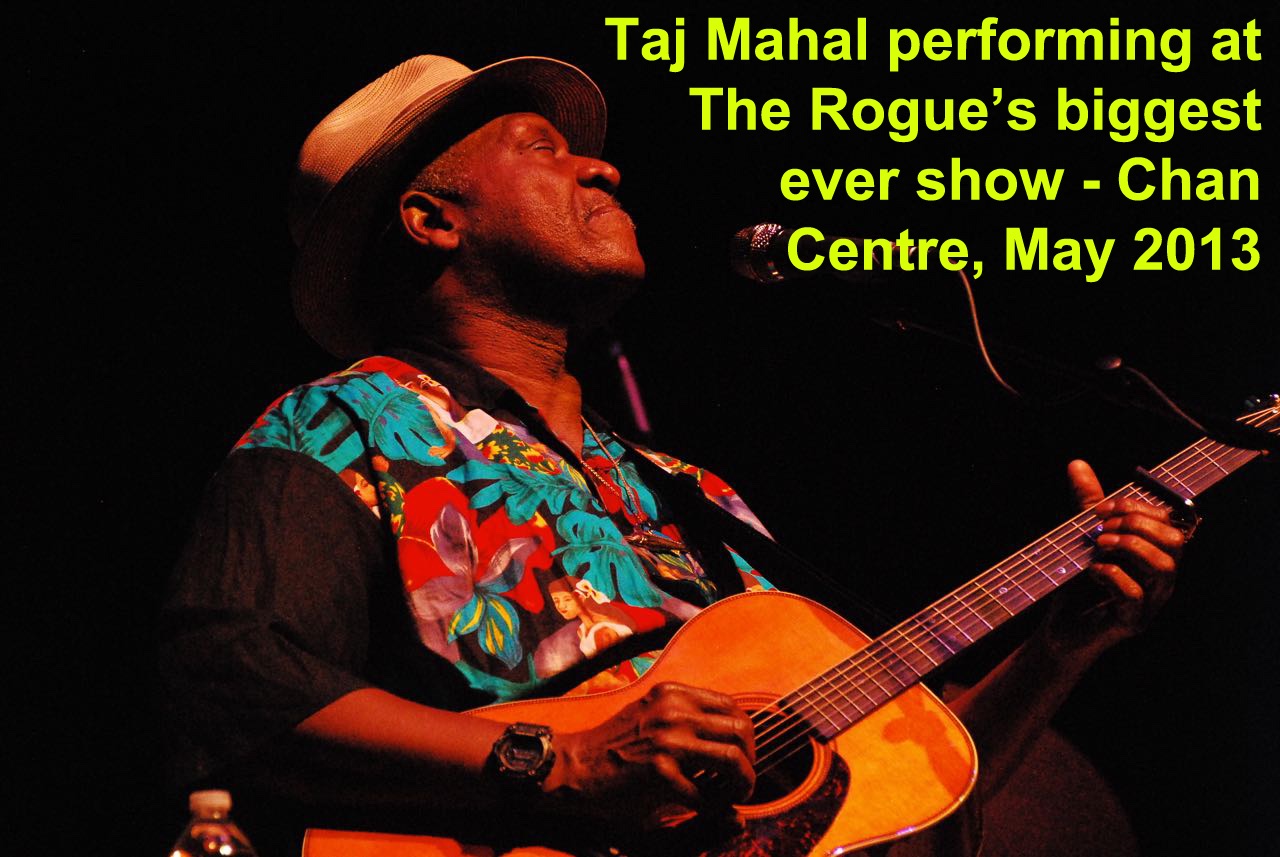The image captures an older Black man, likely in his 60s or 70s, deeply immersed in a musical performance on a dark stage, his face illuminated by the spotlight. He wears a cream-colored fedora and a vibrant shirt with a colorful print featuring luau-like women in grass skirts, leaves, and flowers in hues of blue, red, purple, and pink. His eyes are closed, and his head tilts slightly upward and to the right, suggesting he is lost in the music. In front of him, attached to a stand, is a microphone catching his soulful performance on an acoustic guitar, made of beautifully grained wood. His left wrist sports a black wristwatch, and a water bottle is partially visible at his side. The background is black, emphasizing the performance, with yellow text at the top right corner that reads, "Taj Mahal performing at the Rogue's Biggest Ever Show, Chan Center, May 2013."